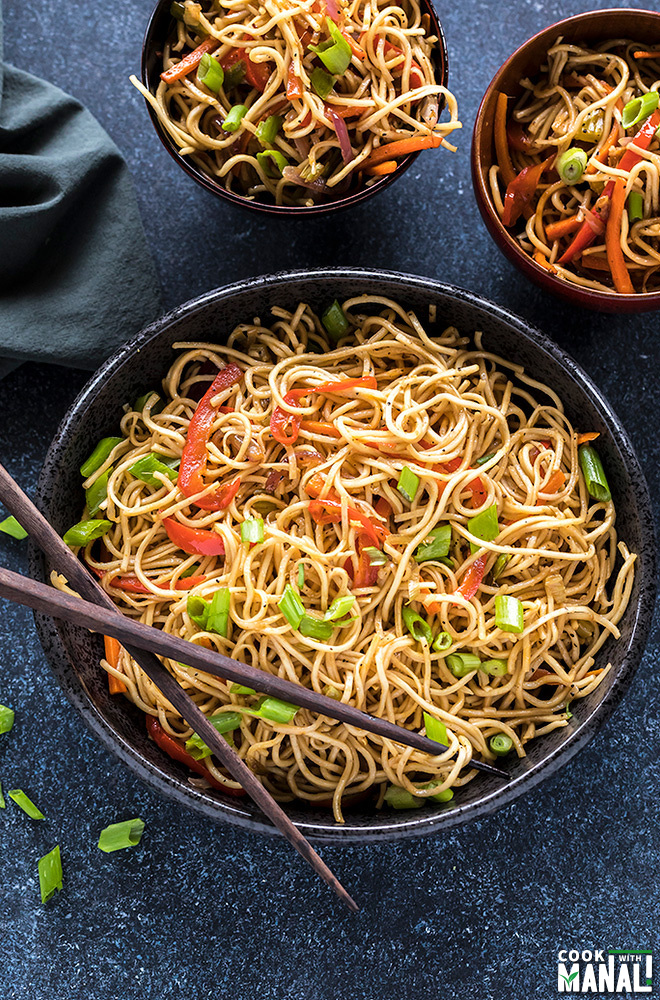The photograph is a vibrant color image showcasing three bowls of chow mein noodles artistically arranged on a dark-colored, possibly stone, blue surface. The shot is taken from above, providing a clear view into each bowl. At the top of the photograph, two smaller bowls, one red and one purple, contain noodles topped with a mix of chopped green onions, carrots, and red peppers. Beneath these, a larger central bowl, dark blue or black in color, holds a more generous portion of chow mein noodles adorned with similar vegetables, including chives and assorted peppers. A pair of chopsticks lies across this large bowl, with one chopstick positioned across the bottom edge and the other resting into the bowl. Scattered around the bowls are a few loose green onions, and on the top left corner of the image, there's a folded black cloth napkin. The bottom right corner of the photograph contains the text "Cook with Manal," indicating a cooking brand or guide.